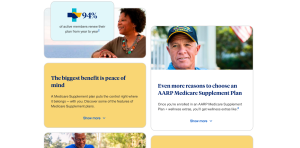The image appears to be a split-screen layout with two distinct sections. The left section is comprised of three content blocks stacked vertically. The top block in this section displays a percentage, "94%", alongside an image of a woman gazing to her left. Directly beneath this is a yellow block with some blue text, although the specifics of the text are not legible. The third block's details on the left side are not mentioned.

The right section contains two blocks. The top block shows a close-up of an older man wearing a hat, which partially extends beyond the upper boundary, cutting off a portion of the hat. The man is facing the camera, but his eyes are directed slightly to the left. Below this image is another yellow block positioned near the bottom, though only the top part of this block is visible and its details are unclear. The overall setting suggests the image is from an AARP website.